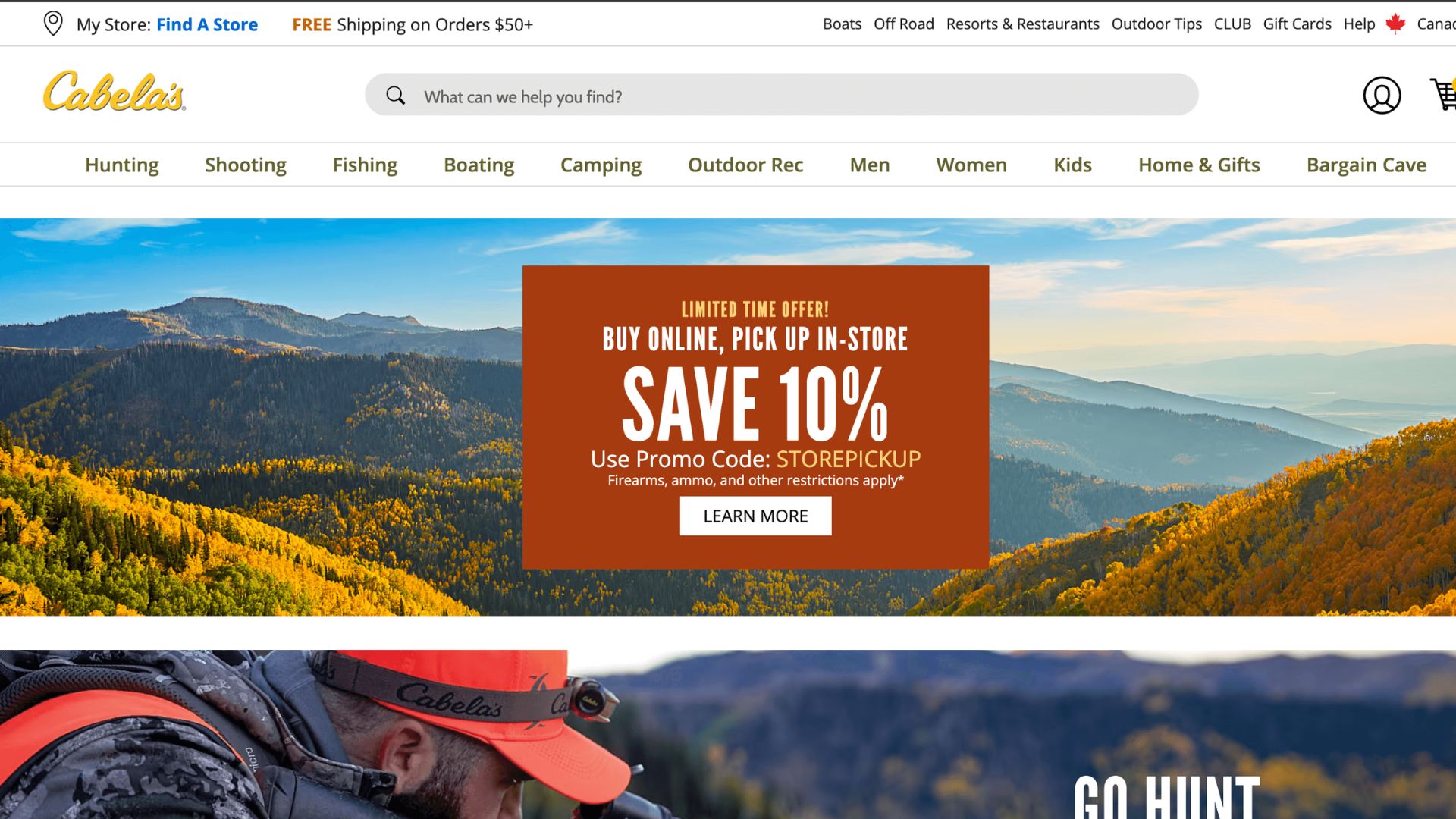This image displays a detailed view of the Cabela's website homepage. In the top left corner, there is a location icon, suggesting the ability to set or view store locations. Just to the right, navigation options include "My Store," "Find a Store," and a banner announcing "Free Shipping on Orders Above $50." Linking to various sections of interest, there are category tabs such as Boats, Off-Road, Resorts and Restaurants, Outdoor Tips, Club, Gift Cards, Help, and Canada.

A central search field prompts, "What can we help you find?" indicating a user-friendly search functionality. The website is identified as being owned by Cabela's, a registered trademark. Underneath the primary navigation, a range of categories is listed, encompassing Hunting, Shooting, Fishing, Boating, Camping, Outdoor Recreational items, as well as sections for Men, Women, Kids, Home and Gifts, and the Bargain Cave.

Prominently featured in the middle is a limited-time offer banner stating: "Buy Online, Pick Up In-Store," and "Save 10% with promo code STORE PICKUP," while noting that certain restrictions apply to firearms, ammo, and other items. A "Learn More" link is available for additional details. 

In the bottom right corner, there is an image of a hunter surrounded by trees, accompanied by a "Go Hunt" call to action, further reinforcing the outdoor and adventure themes central to Cabela's brand.